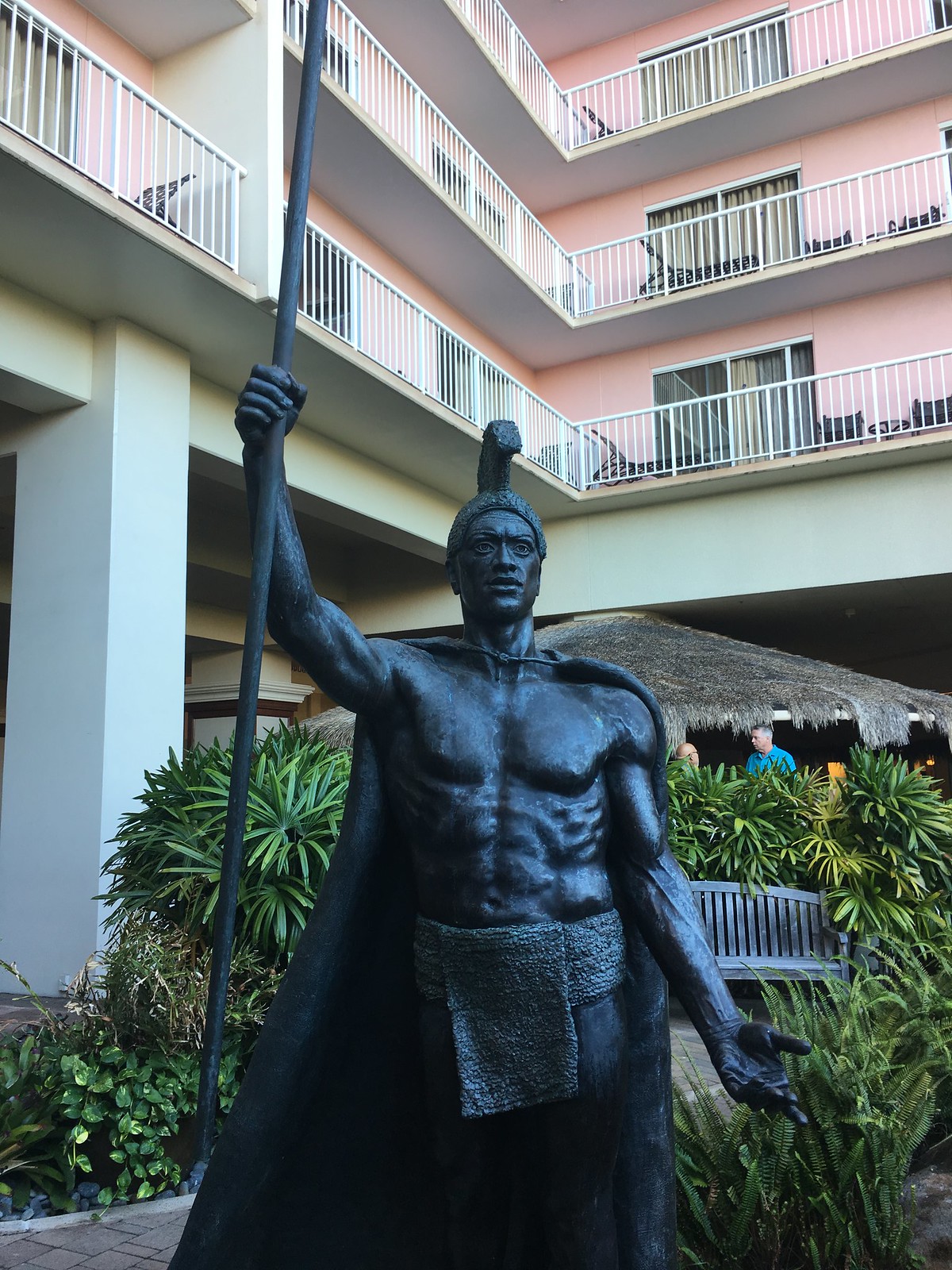The image depicts a large, imposing statue of a fit and muscular Greek man, cast in dark grey or black metal. The statue, positioned in the courtyard of a pink-walled apartment building, shows the man adorned with a helmet and a cape, holding a long stick or spear in his right hand, and wearing a loin cloth around his hips. The apartment building behind the statue features many levels and white fences along the balconies. Additionally, a thatched-roof structure is visible in the background, sheltering two individuals—one of whom is wearing a blue shirt. To the right of the statue, a chair and bench are partially obscured by lush green shrubs that stretch across the backdrop. The scene is rich with greenery, contributing to the overall ambiance of the setting.